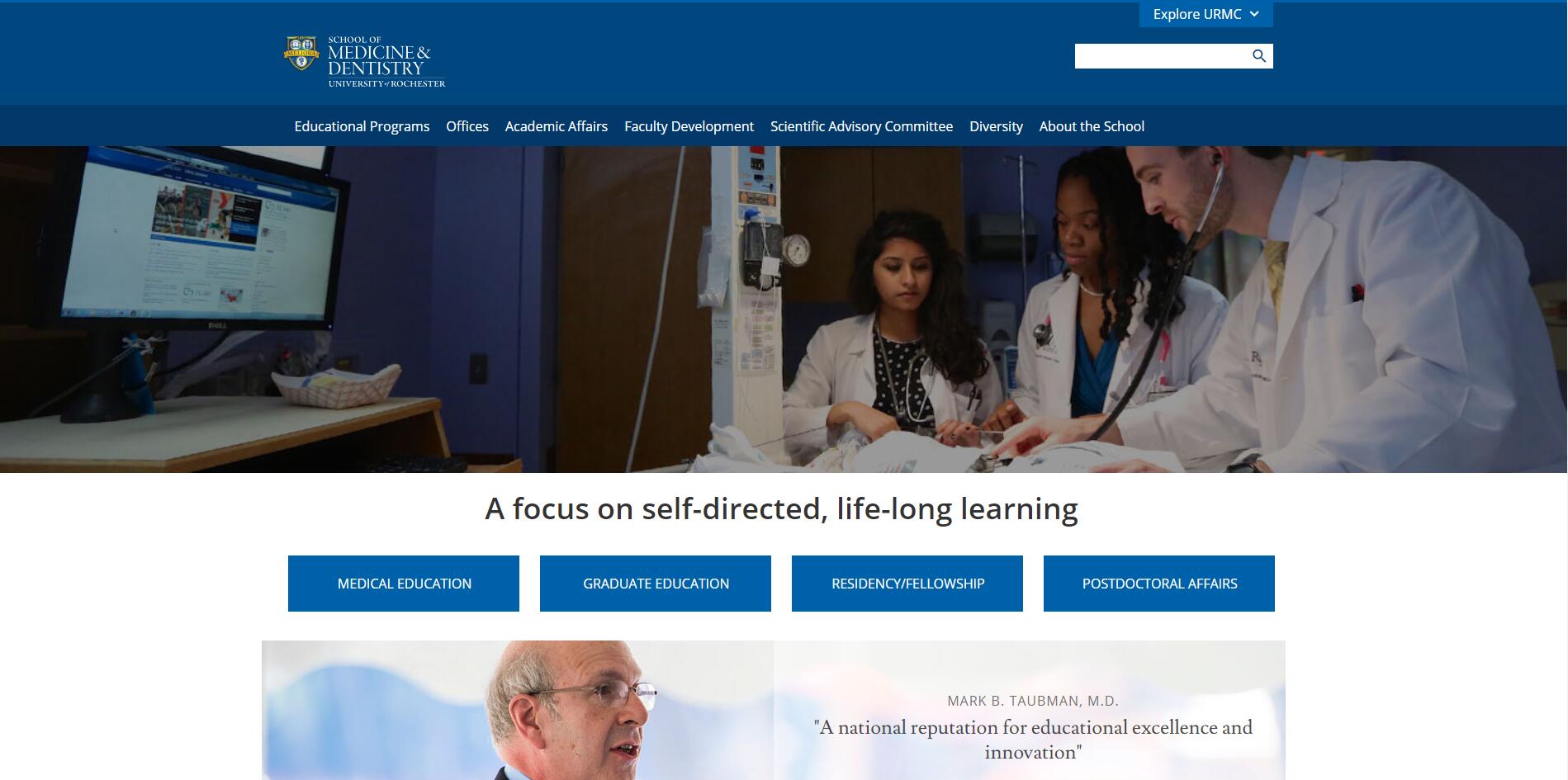This is a screenshot portraying the School of Medicine and Dentistry at the University of Rochester. The image is horizontally oriented, centrally placed on the screen. In the center of the screenshot is a photograph featuring three medical professionals positioned on the right side.

On the far right, a man in a long white coat stands prominently. He wears a yellow and blue striped tie and has dark hair with a bit of stubble on his cheeks and chin. He has a stethoscope in his ears and is leaning towards the left, pressing the instrument against an unseen surface. His stethoscope is silver and black.

To his left stands a dark-skinned woman with long, dark hair that just reaches past her shoulders. She is dressed in a white coat over a blue v-neck top and has a stethoscope draped around her neck. Her body is slightly angled leftward, and she is looking in that direction.

Next to her, on her left, is another woman of shorter stature with long, dark hair cascading over her right shoulder. She has brown skin and is wearing a white coat over a blue and white polka dot shirt. She, too, wears a stethoscope around her neck and is slightly angled rightward, focusing her gaze downward towards the surface where the man is working with the stethoscope.

At the top of the screen, the text reads "School of Medicine and Dentistry, University of Rochester." Centred on the screen is the phrase "A Focus on Self-Directed Lifelong Learning."